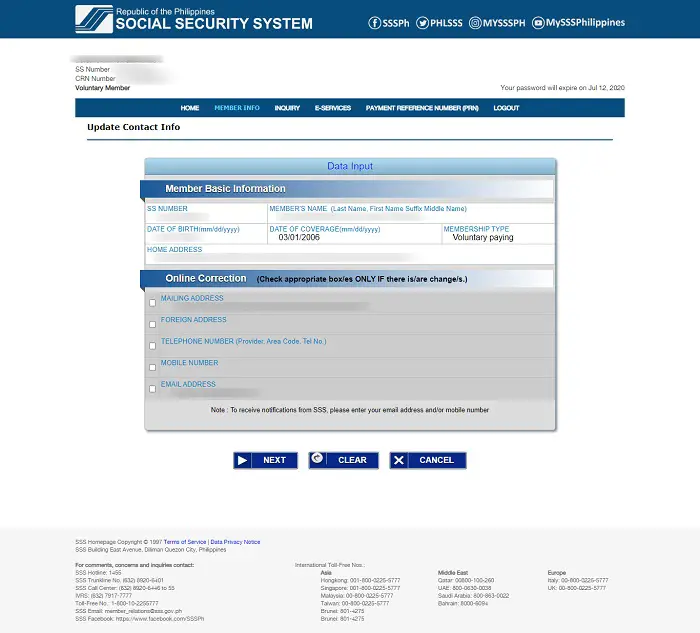This screenshot showcases the homepage of the Social Security System (SSS) website of the Republic of the Philippines. At the top of the page, the SSS logo features three stylized ‘S’ letters arranged in an angular, stacked formation, placed within a white rectangle. Beneath the logo, the text reads "Republic of the Philippines" and "Social Security System."

To the right, social media icons for Facebook, Twitter, Instagram, and YouTube are displayed, each linked to the official SSS accounts, against a blue header background. Below this header, the user's SS number and CRN number are visible but have been blurred for privacy. Additionally, a notice warns the user that their password will expire on July 12, 2020.

The following section contains a navigation bar in a different shade of blue, with menu options like "Home," "Member Info," "Inquiry," "E-Services," "Payment Reference Number PIN," "Logout," and an option to "Update Contact Info." 

The main content area offers fields for data entry titled "Member’s Basic Information," where the user’s name, date of coverage, membership type, date of birth, home address, and SS number are meant to be input but are currently obscured. The section called "Online Correction" includes checkboxes for updating the mailing address, foreign address, telephone number, mobile number, and email address—filled checkboxes are grayed out.

At the bottom of this form are three buttons labeled "Next," "Clear," and "Cancel." The footer of the page displays extensive contact information, including multiple phone numbers categorized by region (Asia, Middle East, Europe), and additional phone numbers for comments and inquiries.